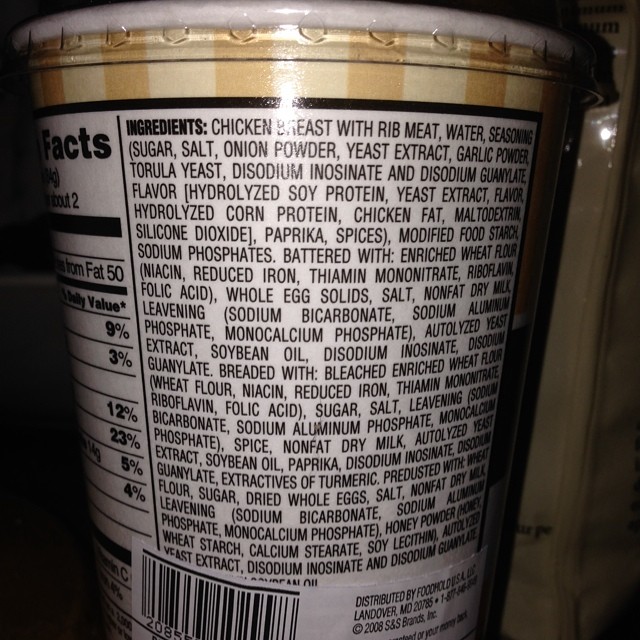Caption: 

The image showcases the ingredient list on the side of a cylindrical container. On the left edge, part of the nutrition facts section is slightly visible, wrapping around the side. The bottom of the container features a white sticker with a barcode and additional information. The top of the container is adorned with a thick striped border in alternating dark gold and light gold colors. Just below this ornate border, the word "Ingredients" is prominently displayed in bold black font. Beneath this header, the ingredients are meticulously listed in smaller, regular black text, extending from the top to the bottom of the container.